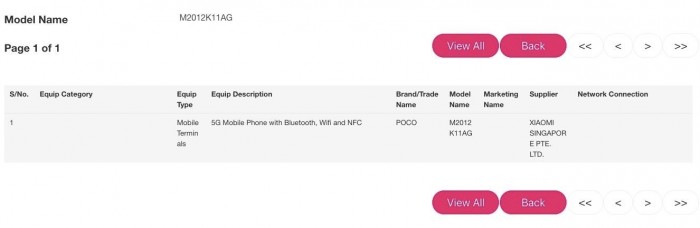This image is a colorful screenshot from an unspecified web page detailing information about a device. At the top of the page, there is a header that reads "Model Name: M2012K11AG, Page 1 of 1". Other navigation options in this header include "View All" and "Back". Additionally, there is a number "1" displayed prominently.

The page classifies the device under the "Equip Category" and "Equip Type" as "Mobile Terminals". The "Equip Description" lists it as a "5G mobile phone with Bluetooth, Wi-Fi, and NFC". The "Brand/Trade Name" is given in uppercase letters as "FOCO". The device's model name is reiterated as "M2012K11AG". 

Notably, the "Marketing Name" field has been left blank, while the supplier is identified as "XIAOMI Singapore PTE Limited". The "Network Connection" field is also blank.

At the bottom of the screenshot, there are two pink oblong buttons. The first button, labeled "View All", has white text. The second button, also with white text, reads "Back". Adjacent to these buttons are four icons contained within smaller white oblong shapes: two arrows pointing to the left, one arrow pointing to the left, one arrow pointing to the right, and two arrows pointing to the right.

The overall format of the screenshot is wider than it is tall, and there are no people visible in the image.